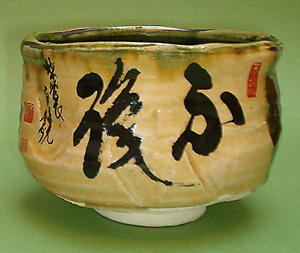This is a detailed photograph of a small, ornamental Japanese ceramic cup, possibly a teacup or bowl. The cup is predominantly a beige or yellowish color with intricate black and red calligraphy-style Japanese characters adorning its exterior. On one side, a character resembling a scribbled "K" is followed by another character that looks like a "D" with an attached dash and post, accompanied by a small red rectangular piece to its right. Behind the left character is additional writing in black ink. The top rim of the cup is a green hue, and the inside may share this green color. The base is white and unglazed, providing a contrast to the glazed exterior. The cup sits on a green surface, casting a shadow, and the photograph highlights its handcrafted, slightly irregular form, reminiscent of a beginner's pottery piece, yet maintaining its unique aesthetic charm.